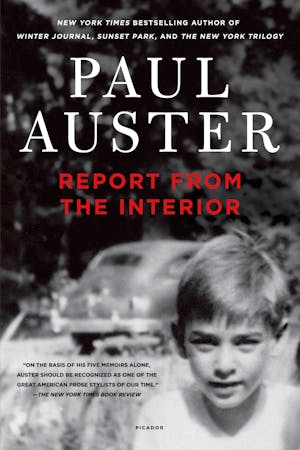The book cover features a vintage black and white photograph set against a black or grey background. Dominating the bottom right corner, a boy with smooth, blondish hair, wearing a white shirt, gazes directly into the camera. Behind him, a grey, vintage car, suggestive of the 1940s or 50s, drives away, adding to the nostalgic atmosphere. The backdrop also includes trees at the top of the image, enhancing the retro feel. Above the photo, in white text, the cover highlights "New York Times bestselling author of Winter Journal, Sunset Park, and the New York Trilogy." The author's name, "Paul Oster," is prominently displayed in a large serif font. Beneath, in striking red font, "Report from the Interior" announces the book's title. Additionally, there's a testimonial in black font from the New York Times which reads, "On the basis of his five memoirs alone, Oster should be recognized as one of the great American prose stylists of our time."